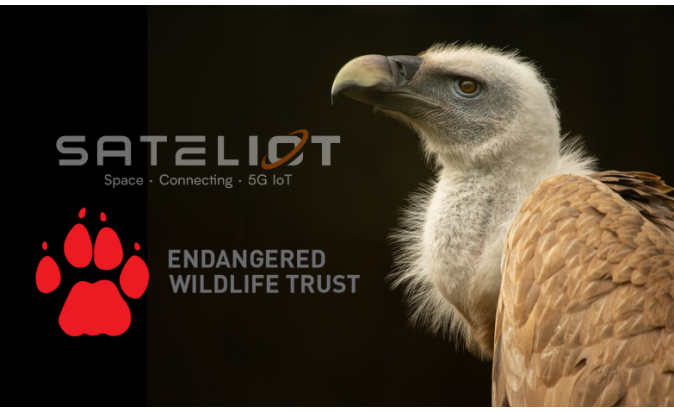In this horizontally aligned rectangular image with digital enhancements, a striking profile of a bird, likely an eagle, dominates the right half against a solid black background. The bird's distinct features include a tall, curved beak similar to a parrot's, a white head, white-grayish face and neck, dark brown wings with lighter brown feathers, and dark brown-reddish eyes, although only half of its body is visible. The left side of the image features prominent text. At the center-left, in large gray capital letters, "SATELLIOT" is displayed, with a ring circling the "O." Below it in smaller gray letters, it reads, "SPACE CONNECTING 5G-IOT." Further down, a red paw print signifies the "ENDANGERED WILDLIFE TRUST," written adjacent in gray all caps. The overall composition juxtaposes the bird's vibrant natural details with the stark, black digital background, enhancing the focus on the bird and the important messaging.